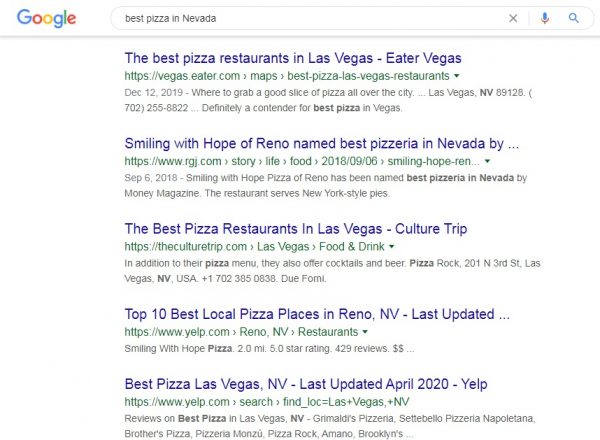This image is a detailed screenshot of a Google search page with a white background. In the upper left corner, the Google logo is displayed in its signature color scheme: the capital 'G' is blue, the first 'o' is red, the second 'o' is yellow, the lowercase 'g' is blue, the 'l' is green, and the 'e' is red. To the right of the logo is a search bar with the query, "Best Pizza in Nevada," typed in it. Adjacent to the search bar are three icons: an 'X' for clearing the search, a microphone for voice search, and a magnifying glass for initiating the search.

Below the search bar, five search results are displayed. The first result is titled "The Best Pizza Restaurants in Las Vegas," from Eater Vegas, dated December 12, 2019. Its description reads, "Where to grab a good slice of pizza all over the city," and is followed by the location "Las Vegas, Nevada," the postal code "89128," and a phone number claiming it as a contender for the Best Pizza in Vegas.

The second result features "Smiling with Hope of Reno, named Best Pizzeria in Nevada," partially obscured by an ellipsis, and provides a web address. It states that "Smiling with Hope Pizza of Reno has been named Best Pizzeria in Nevada by Money Magazine," and is known for serving New York-style pies.

The third result, "The Best Pizza Restaurants in Las Vegas," from Culture Trip, includes a web address and mentions that in addition to their pizza menu, these establishments also offer cocktails and beer. "Pizza Rock" at "201 North 3rd Street, Las Vegas, Nevada, USA" and a phone number are also mentioned.

The fourth result lists "Top 10 Local Pizza Places in Reno, Nevada." The web address and the establishment "Smiling with Hope Pizza" are mentioned but no additional details are visible.

The fifth result is for "Best Pizza in Las Vegas, Nevada," last updated in April 2020 from Yelp. It provides a web address and reviews for various pizzerias, including "Grimaldi's Pizza," "Cetabello Pizzeria in Napatana," "Brothers Pizzeria in Monsieu," "Pizza Rock," "Amano," and "Brooklyn's."